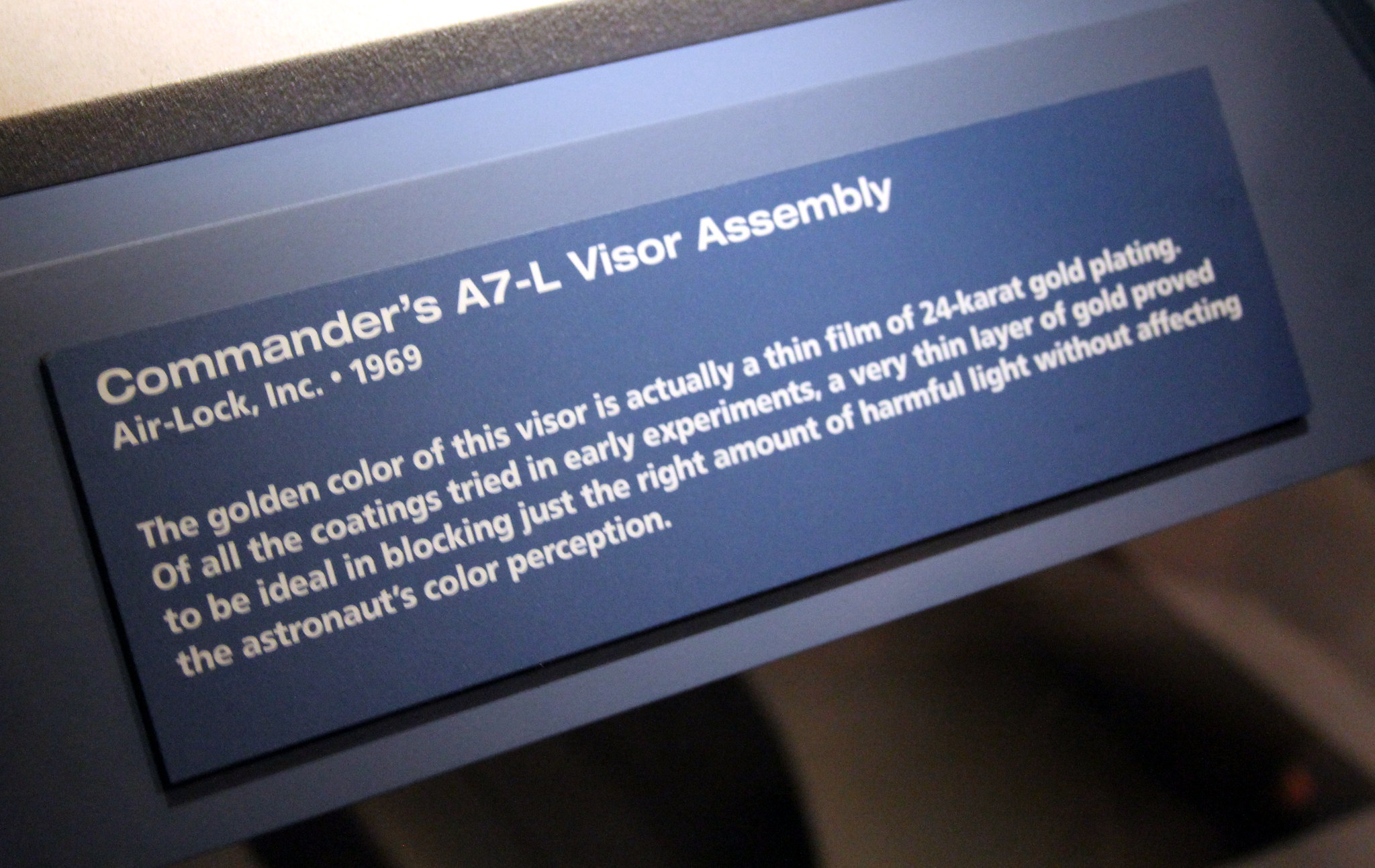The image captures a detailed photograph of a museum sign, which is a horizontal rectangle in shape, photographed at a diagonal angle. The sign itself, a plaque, is predominantly blue with various shades and layers ranging from light blue to dark blue, creating a gradient effect. Centered within this blue plaque is a panel with six lines of white text. The top line reads "Commander A7-L Visor Assembly," followed by "Airlock, Inc, 1969." Below these, a descriptive paragraph explains that "The golden color of this visor is actually a thin film of 24 karat gold plating. Of all the coatings tried in early experiments, a very thin layer of gold proved to be ideal in blocking just the right amount of harmful light without affecting the astronaut's color perception." The background behind the plaque features colors like gray, dark gray, black, white, and beige. The overall setting suggests an indoor museum exhibit or a gallery display, likely within an aerospace or astronautical context.